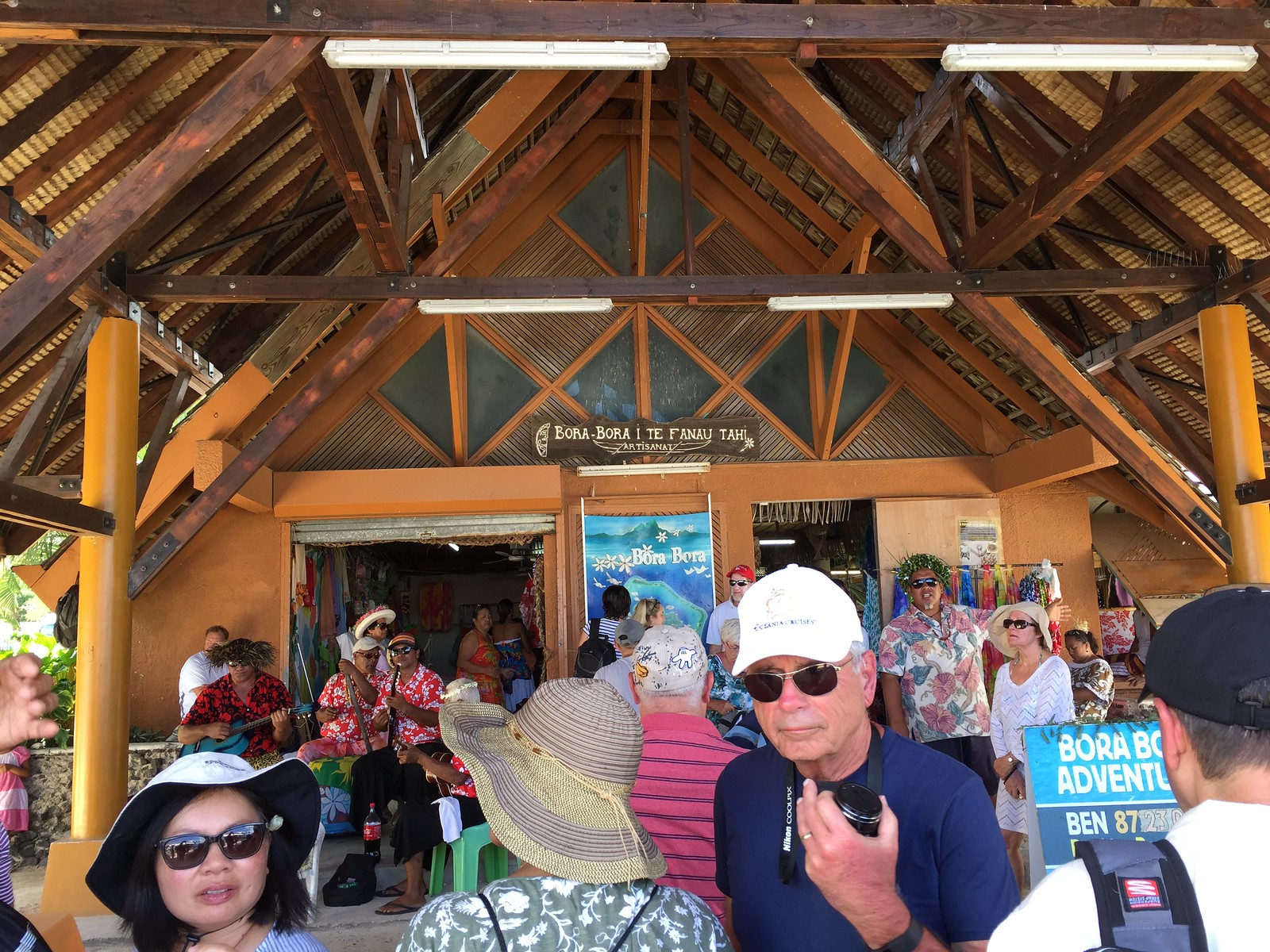This photograph captures an outdoor event under a covered A-frame structure adorned with wooden beams and rafters. The venue, associated with Bora Bora, features multiple signs: one sign reads "Bora Bora Aite Fanu Tai" in yellow carved letters and another states "Bora Bora Adventures." An open, garage-style door on the left reveals trees in the distance, further suggesting an outdoor recreational scene. The gathering comprises over a dozen people, predominantly wearing summer hats and sunglasses, with many dressed in floral, Hawaiian-style shirts indicative of a warm, tropical climate. Amongst the crowd, a man in the middle wearing a white hat, sunglasses, and a blue t-shirt holds a camera, while a woman in the bottom left corner also sports a white hat and sunglasses. To the left of the image, a small band performs, with members dressed in red and white floral shirts and one musician playing a blue guitar. The ambiance is casual and vibrant, resonating with the spirit of a tropical getaway.